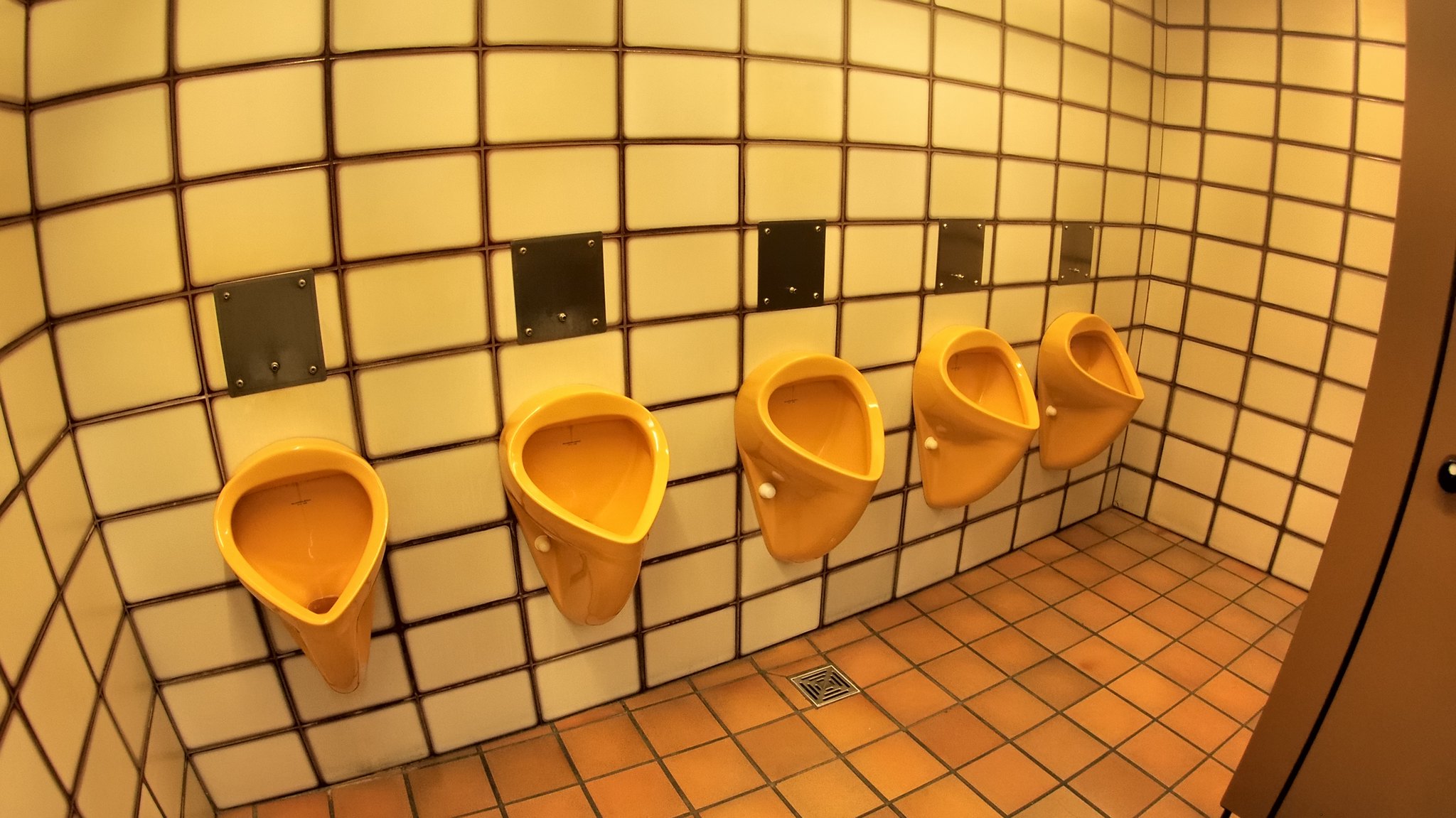The image depicts a contemporary men's public restroom captured with a fisheye lens, which gives the photo a bubbled and distorted appearance. There are five identical yellow-golden urinals mounted on a wall covered in large rectangular yellow tiles with dark brown grout. Each urinal has a stainless-steel panel with a small flush button above it. The floor is tiled with terracotta-colored square tiles, also grouted with dark brown mortar. Directly below the central urinal, there is a small square floor drain. In the foreground, the lower left corner reveals part of a tan wall and a doorway, suggesting the presence of another section or entry point within the restroom.